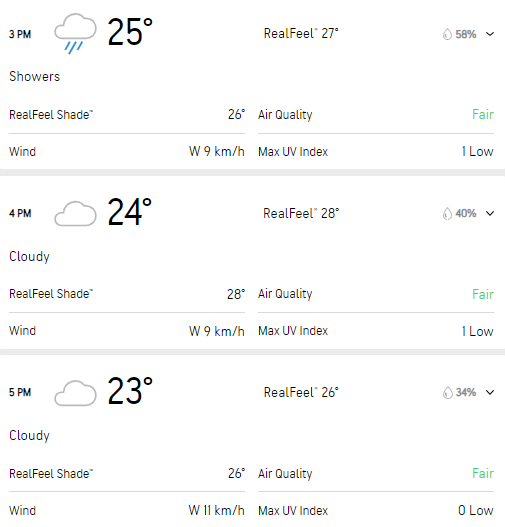Detailed Weather Website/App Screenshot Description:

The image captures a screenshot of a weather website or app featuring a clean white background with predominantly black text and some green text on the far right. The display is divided into three sections, each providing detailed weather information for consecutive hours.

Starting at the top, the time is indicated as 3 p.m. Accompanied by an icon depicting a cloud with rain, the weather condition is labeled "Showers." The temperature is recorded at 25 degrees Celsius with a "RealFeel" temperature of 27 degrees. Additional details include a 58% chance of rain, a RealFeel shade temperature of 26 degrees, and an air quality rating of "Fair." The wind speed is noted to be 9 kilometers per hour coming from the west, and the maximum UV index is marked as 1 (low).

The next section details the weather for 4 p.m., showing a temperature of 24 degrees Celsius under "Cloudy" conditions. The chance of rain stands at 40%, with a RealFeel temperature of 28 degrees and a RealFeel shade temperature of 28 degrees as well. The air quality remains "Fair," and the wind continues to blow from the west at 9 kilometers per hour. The maximum UV index is still 1 (low).

The final section provides the forecast for 5 p.m., indicating "Cloudy" weather with a temperature of 23 degrees Celsius. The RealFeel temperature is 26 degrees, with a 34% chance of rain and a RealFeel shade temperature of 26 degrees. The air quality persists as "Fair," but the wind speed increases slightly to 11 kilometers per hour, coming from the west. The maximum UV index drops to 0 (low).

This comprehensive layout offers a clear and detailed snapshot of the weather conditions, including temperature variances, precipitation chances, air quality, wind speed and direction, and UV index for the given times.